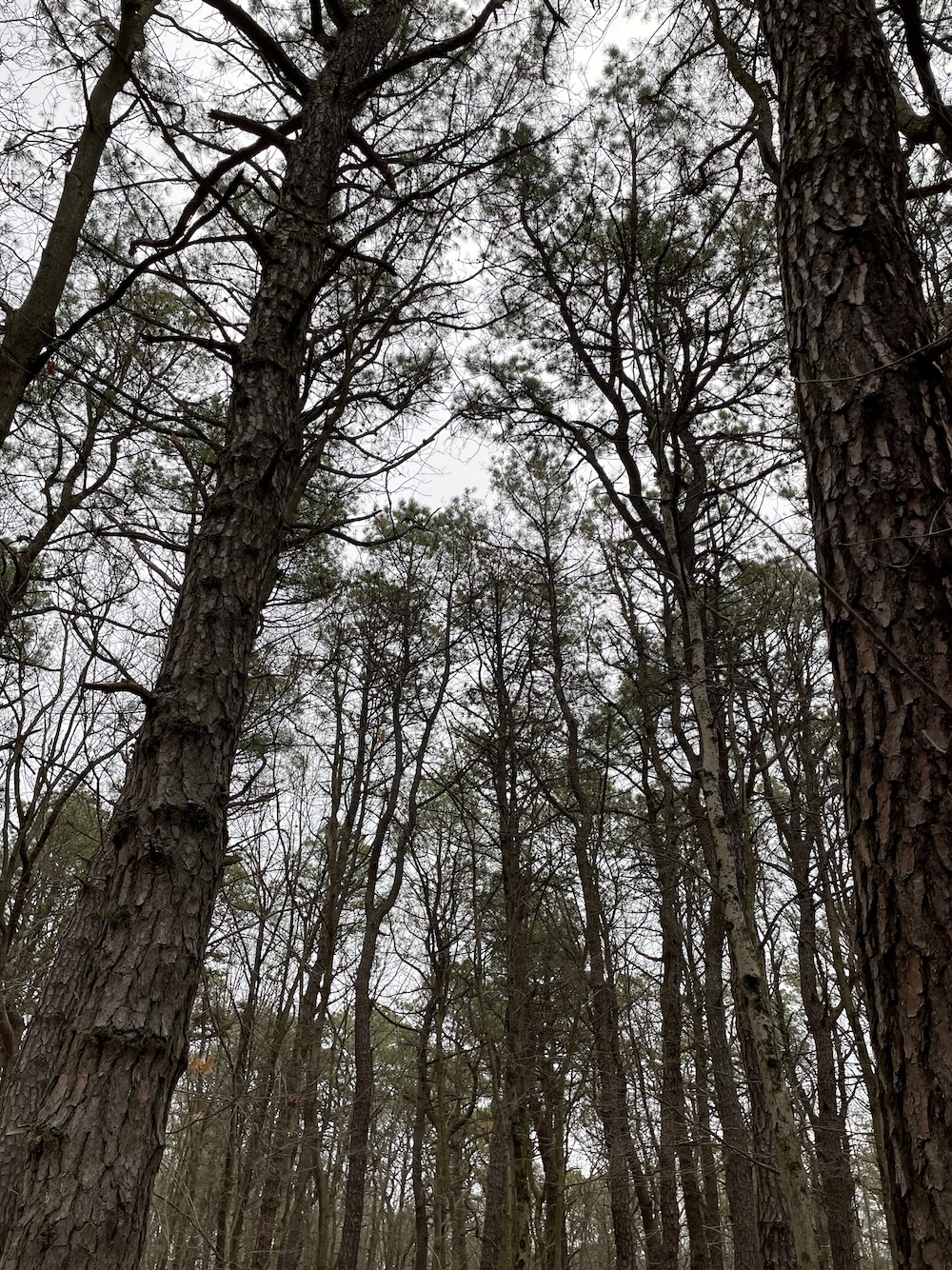The image captures a dense forest scene during what appears to be the fall season, as the remaining foliage is sparse with minimal greenery. The focus is on tall, slender trees with varying bark patterns, ranging from black and lighter gray vertical strips to predominantly white sections. These trees, likely pine or a similar species, have very few lower branches and stretch high into an overcast sky heavy with either clouds or the arrival of rain. The vantage point is from the forest floor looking upwards, emphasizing the towering trunks and the canopy far above, giving the impression of numerous lines pointing towards the bleak, white-gray sky.